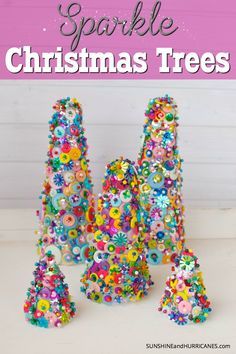The image is a small, rectangular photograph featuring a colorful, crafty scene. At the top, the background is purple, adorned with white sparkling dots, and it bears the word "Sparkle" in gray, silvery letters. Below that, "Christmas Trees" is prominently displayed in bold white letters. The central section of the image showcases five uniquely decorated Christmas trees arranged in a playful manner: two at the back, one in the middle, and the remaining two towards the bottom right. These trees are creatively constructed from various objects resembling circular pins, knick-knacks, or fabric pieces, all glued together. They boast a vibrant array of colors, including yellow, purple, white, green, red, and blue. The trees sit on a white surface against a backdrop of white wood paneling. At the bottom right corner, the website "sunshineandhurricanes.com" is visible in black text, albeit slightly blurry.